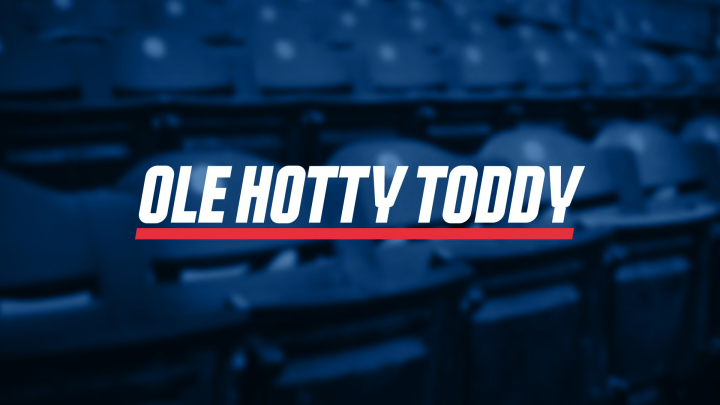The image features a horizontal orientation with a background of what appears to be rows of blue, plastic seats, similar to those found in a stadium or on bleachers. The background is indistinct and somewhat blurry, creating a dark blue ambiance that is lighter towards the top center and darker at the corners. Central to the image is a bold, white, italicized text in a sans-serif font that reads "O HOT TOTTIE," with the text underlined in red. The top surface of the seats reflects light, revealing their rounded contours. The image seems to function as an advertisement, possibly for a brand related to food, set against this stadium-like backdrop.